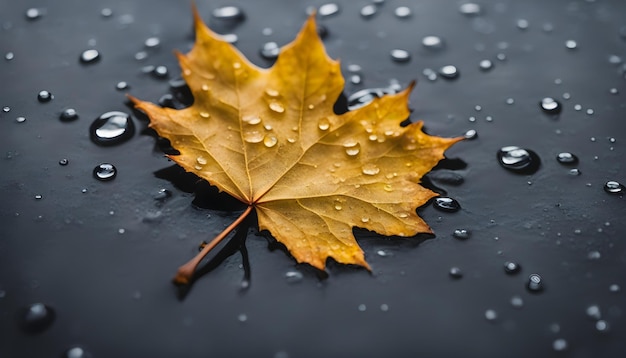The photograph is a hyper-realistic, outdoor shot taken during the daytime. The rectangular image, approximately four inches wide by two to three inches high, features a striking contrast between its dark gray, almost black, painted cement background and the golden-brown maple leaf positioned slightly off-center. The background, made to look like smooth, worn metal or plastic, is speckled with water droplets of varying sizes, suggesting a recent rain shower. These droplets are scattered across both the leaf and the surface, gradually fading into a blur near the image’s corners, thus drawing the viewer’s focus towards the center. The maple leaf, with its five defined lobes, reveals intricate vein patterns and is still attached to its thin, red-brown stem, which points towards the lower left of the image. The high clarity of the photograph emphasizes the texture and color variations, making the leaf appear almost three-dimensional against the sleek, moist surface.